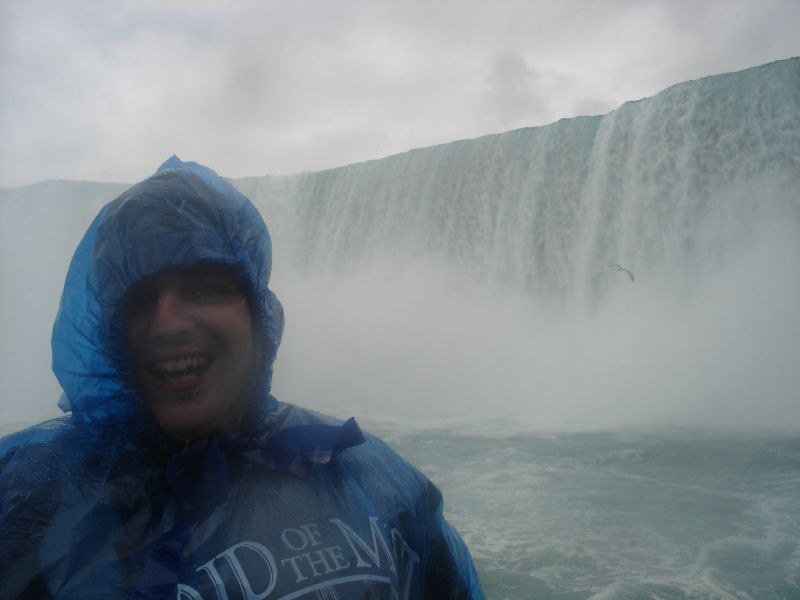The photograph captures a person, likely a woman, standing on the left side of the frame, with the upper third of the image showcasing a backdrop of gray skies. She is smiling broadly, though her face is partially covered by the hood of a blue, semi-transparent raincoat inscribed with the words "Maid of the Mist" in white letters—a clear reference to the popular boat tour at Niagara Falls. The majestic waterfall occupies the distant background, stretching across the entire width of the image and generating a thick mist that envelops the scene. Beneath the waterfall, the water appears churned and tumultuous, displaying shades of greenish-blue. It’s unclear whether the person is standing on a boat or on land. The confluence of mist, swirling waters, and overcast skies adds a dramatic and atmospheric quality to the photo.